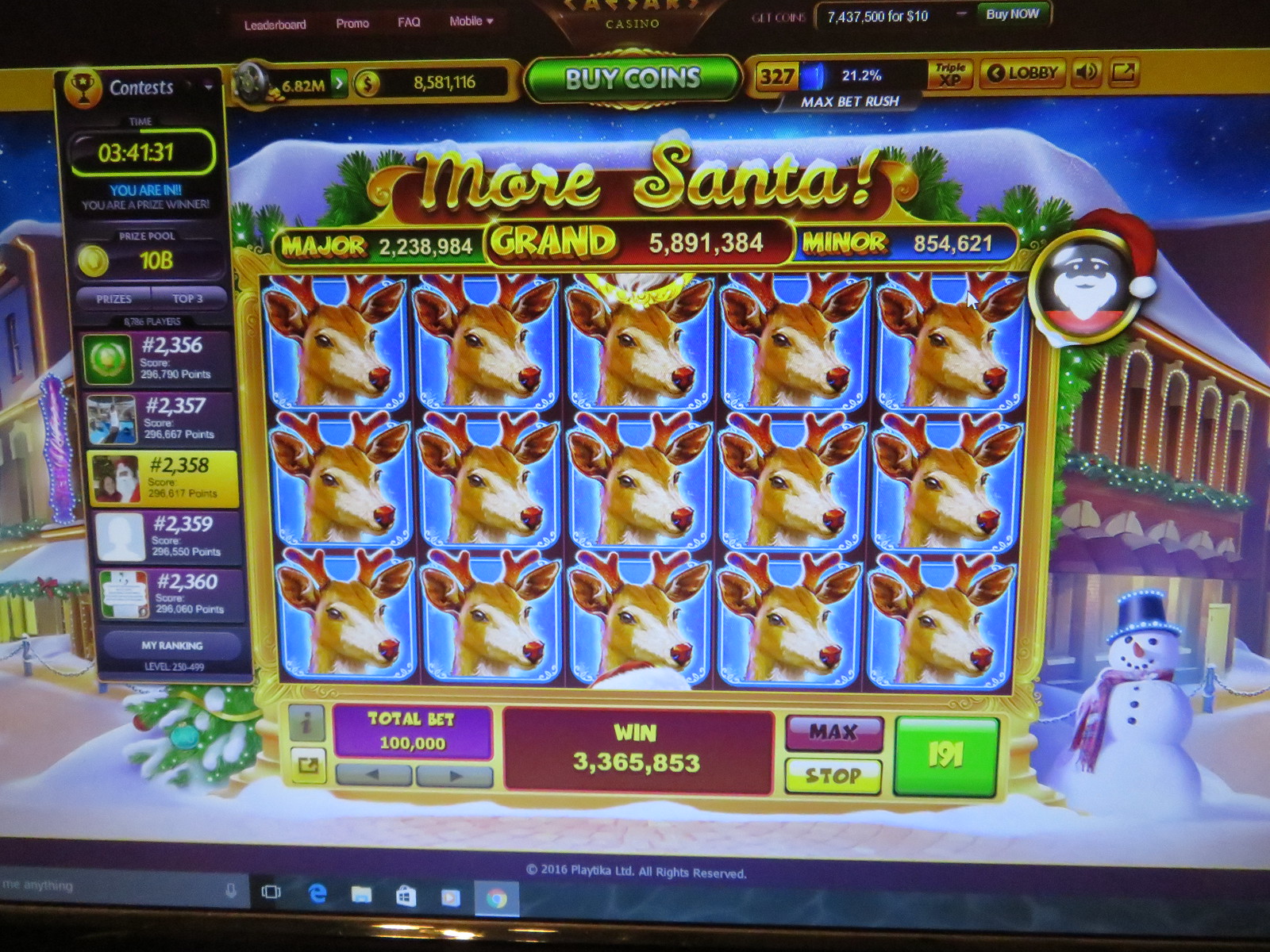The image captures a screenshot of a festive, Christmas-themed online slot machine game running on a Windows 10 or 11 operating system. The main screen prominently displays the title "More Santa!" in gold at the top. The interface features a traditional casino layout, with the word "casino" centrally located in the top menu. To the left of the menu, various options and a leaderboard are visible, displaying different player metrics, including a timer and scores.

In the center of the screen is a 5x3 grid, totaling 15 slots, each filled with a light brown reindeer with a darker brown nose, indicating a winning combination. The left sidebar includes a leaderboard, showing the player in third place. Above the reindeer grid, major and grand jackpot amounts are listed, with figures such as $2,238,984 and $5,891,384, respectively.

A win summary at the bottom notes a total bet of $100,000 and a massive win of $3,365,853. The background complements the theme with a Christmas aesthetic, featuring a snowman, a Christmas tree, snow-draped buildings, and holly decorations, creating a festive North Pole ambiance. The right side of the screen includes options for buying more coins and showing current scores.